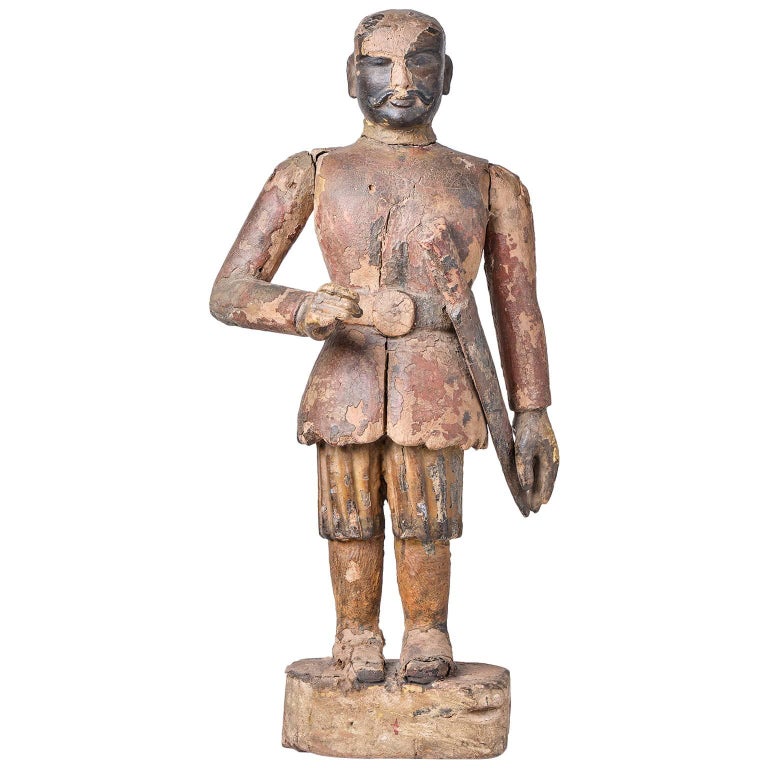This photograph depicts a highly weathered, antique statue of a soldier, standing against a plain white backdrop. The statue, potentially crafted from clay or terracotta, bears a reddish-brown color with various shades of brown and splotches of what appears to be reddish corrosion. The figure exhibits signs of aging, with much of the original paint chipped off.

The soldier is adorned in attire that suggests an ancient or possibly 1700s era, featuring a long-sleeved jacket that has largely lost its dark red hue, and a pair of pants or britches that end just above what seem to be shoes or boots. He sports a prominent mustache and appears to have a bald or minimally-haired head, with noticeable impressions of his eyes and facial features, indicating significant wear.

A large belt with a circular buckle secures his coat, and from this belt hangs a sword or sheath, running down his left side almost to his knee. Notably, the sword has a red handle and looks weathered, blending with the overall aged appearance of the statue. The soldier's right hand is bent in front of him, while his left arm hangs straight down by his side. The statue stands on a short cylindrical pedestal, further contributing to its ancient, possibly artifact-like aura. Overall, the statue encapsulates an image of a time-worn soldier, suggesting a rich historical past.